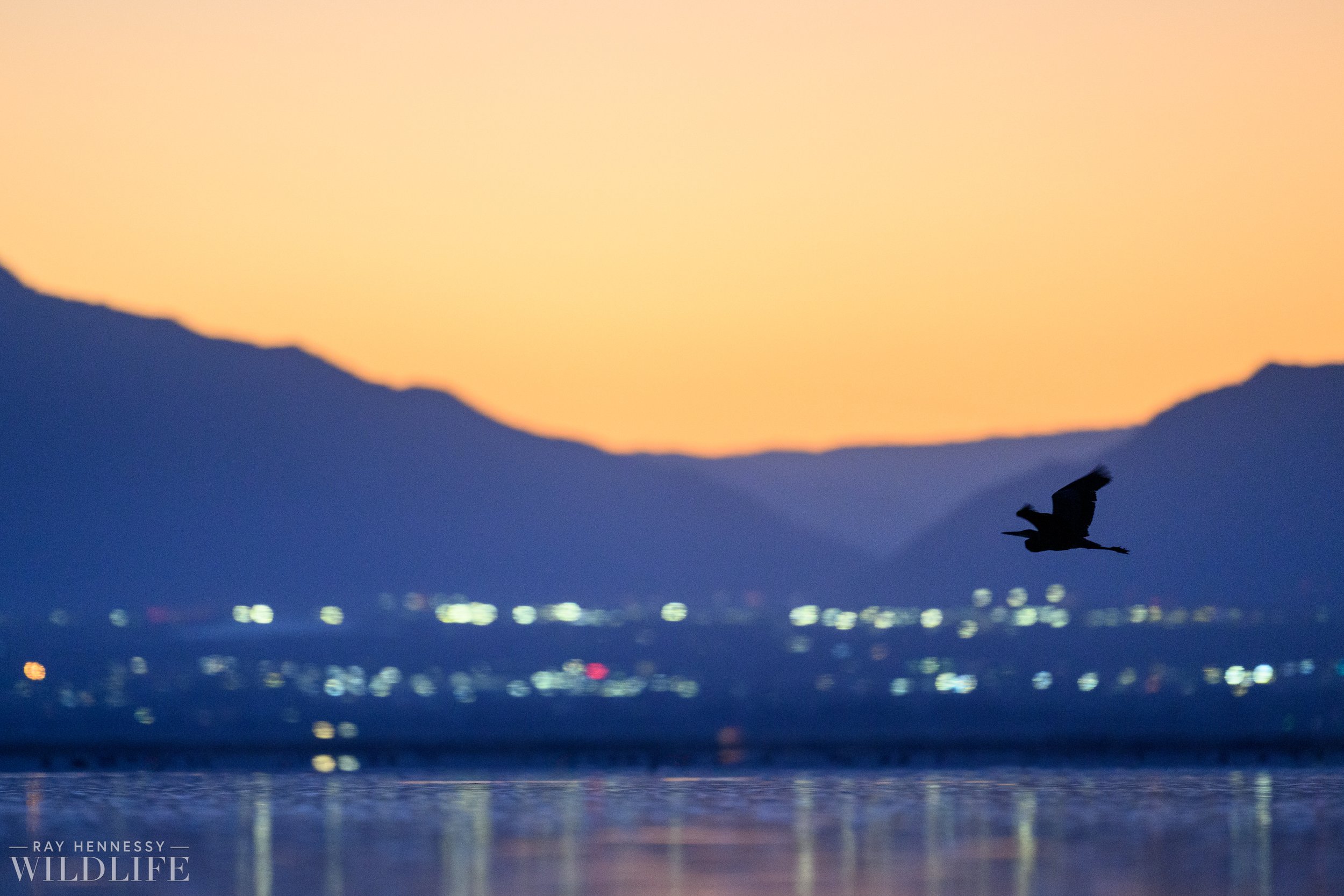This stunning wildlife photograph by Ray Hennessy captures a serene and picturesque evening scene. In the bottom left corner, the photograph is attributed to Ray Hennessy Wildlife. Dominating the background is a breathtaking orange and pink sunset that bathes the landscape in warm hues. Just below the vibrant sky, you can see a trio of mountains, with two closer to the foreground and one in the distance. The city lights beneath the mountains are slightly out of focus, creating a magical, twinkling effect that stretches across the entire width of the photo. These lights reflect off the tranquil water below, adding to the scene's enchanting ambiance. In the middle of the frame, a small to medium-sized bird is captured in silhouette as it flies from right to left over the still water, adding a dynamic element to the otherwise peaceful setting. The deep purplish mountains and the bright, colorful sky together make this photograph an evocative and beautiful portrayal of nature's quiet moments.